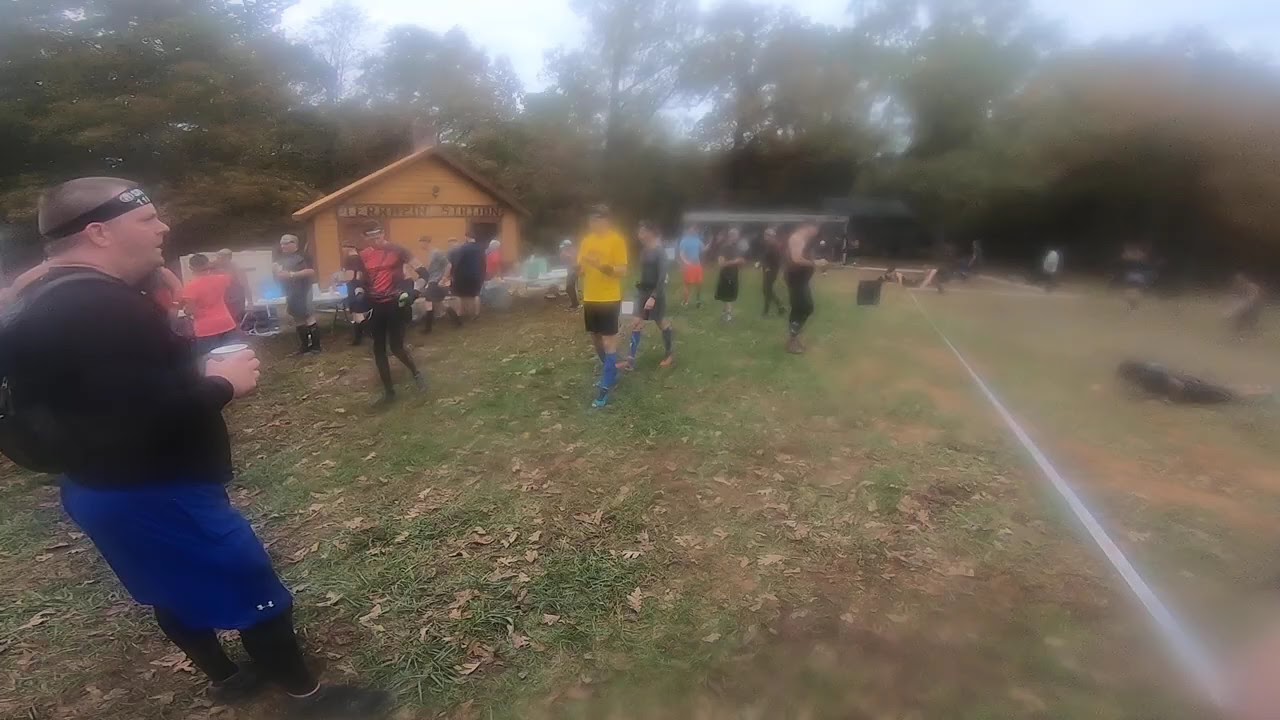In this extremely blurry image, taken outdoors, a group of people is gathered at what appears to be a sporting event or some sort of competition. The scene is set on a grassy area, possibly a park, with a white stripe running along the ground that might designate a playing field. It's somewhat rainy, as water droplets seem to have affected the lens quality. On the left lower part of the image, there's a heavyset man who stands out clearly, wearing a black jacket, blue shorts with dark leggings underneath, dark tennis shoes, and a black headband. He's holding a white cup, possibly containing a beverage. The people in the crowd are mostly dressed in running gear, headbands, and shorts, suggesting they are participants in the event. In the background, there are indistinct, blurry trees and sky, along with an orange A-frame building with an unreadable sign, adding depth to the scene. Despite the blurry quality and the out-of-focus faces, the image captures the essence of a community gathering or athletic event under potentially cloudy skies.